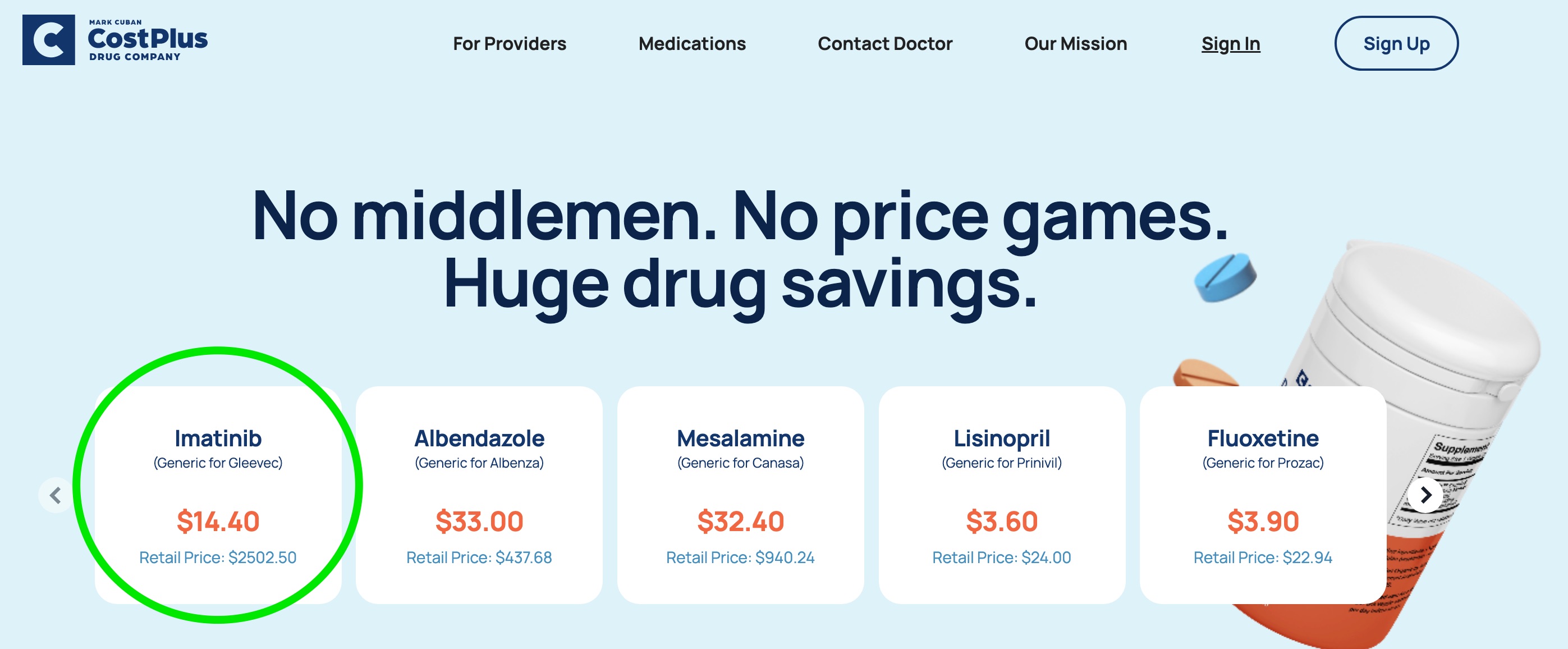### Caption:

The image depicts the COSPLUS Drug Company website with branding that prominently features a C in light blue on a dark blue background in the top left corner. The navigation bar at the top provides various options including "For Providers," "Medications," "Contact Doctor," "Our Mission," "Sign In," and a bright sign-up button. The website background is a very light blue, maintaining a clean and user-friendly interface. 

Central to the image is a bold statement: "No Middleman, No Price Games, Huge Drug Savings," emphasizing the company's mission to provide affordable medication.

Below this statement, there are five detailed product boxes displaying drug information. The first box highlights **Imatinib (generic for Gleevec)**, with a price of $14.40 in orange contrasted against a retail price of $2,502.50 in blue.

The second box presents **Albendazole (generic for Albenza)**, priced at $33.00 with the retail price marked at $437.68.

The third box features **Mesalamine (generic for Canasa)**, listed at $32.40, significantly lower than its retail price of $940.24.

Overall, the image effectively communicates the considerable cost savings provided by COSPLUS on essential medications, illustrating their commitment to affordability and transparency.